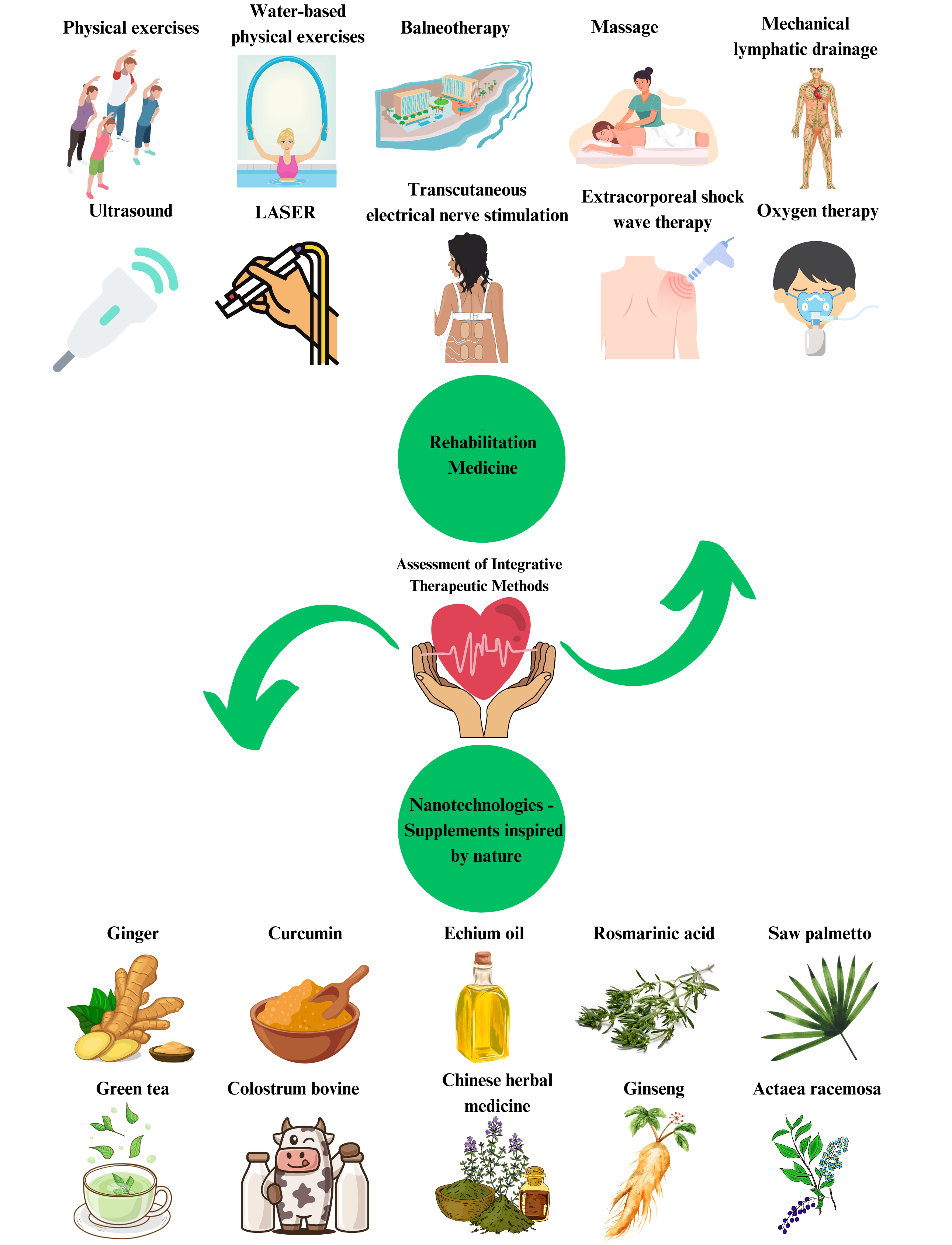The illustrated graphic is a detailed and colorful flowchart depicting various integrative therapeutic methods. At its center, a pair of hands cradles a light pink heart adorned with a heart rate illustration, with two green arrows on either side—one curving upwards to the right, and the other curving downwards to the left. The text above the heart reads "Assessment of Integrative Therapeutic Methods." Atop the graphic sits a green circle labeled "Rehabilitation Medicine," beneath which are ten icons representing different medicinal options: physical exercises (illustrated by four people stretching), water-based exercises (a woman in a pool with a noodle), balmy-o therapy (a beachfront massage scene), medicinal mechanical lymphatic drainage (a human body chart), ultrasound, laser, transcutaneous electrical nerve stimulation, extracorporeal shockwave therapy, and oxygen therapy. 

Below the central heart graphic is another green circle that says "Nanotechnologies Supplements Inspired by Nature," featuring vivid hand-drawn illustrations of ten herbal and plant-based supplements, including ginger, curcumin, ecchium oil, rosmarinic acid, saw palmetto, green tea, colostrum bovine, Chinese herbal medicine, ginseng, and Actaea racemosa. The entire diagram serves as an educational tool that contrasts rehabilitation medicine with nanotechnology-driven, nature-inspired supplements, using engaging cartoonish illustrations to visually explain each modality.